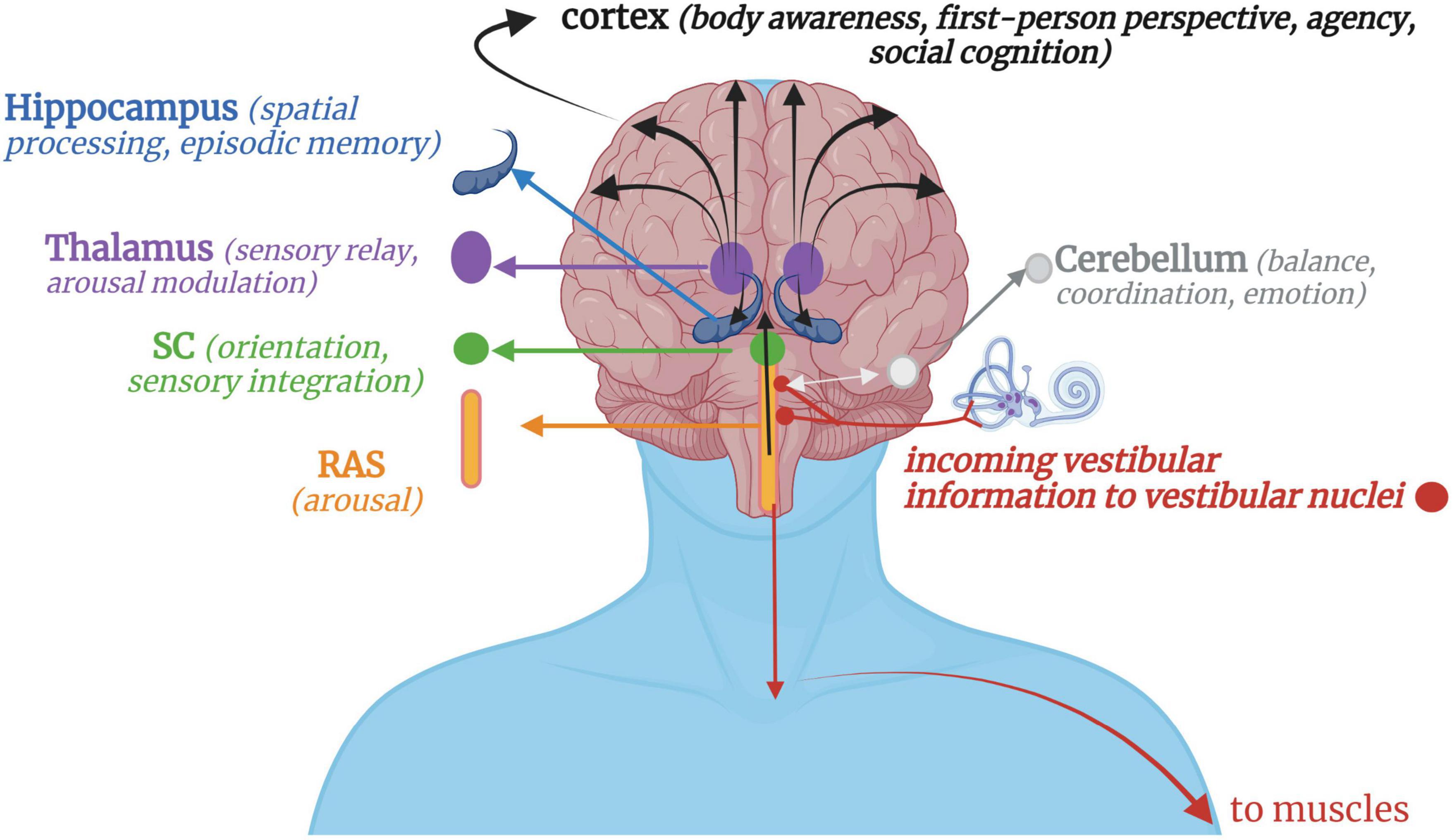The image is an illustrative and detailed diagram of a brain with a blue silhouette of neck and shoulders. The brain, depicted in a large, pink form covering the entire head, highlights various anatomical regions and their functions for educational purposes. Multicolored arrows and circles—black, purple, green, red, blue, and yellow—point to different brain parts such as the cortex, hippocampus, thalamus, cerebellum, and structures involved in sensory integration and arousal. Notable features include purple dots in the middle, blue objects below, a green circle, a yellow line, and red lines and arrows indicating connections to muscles. Descriptions like sensory relay, spatial processing, and arousal modulation accompany these regions, emphasizing the detailed and informative nature of the graphic.